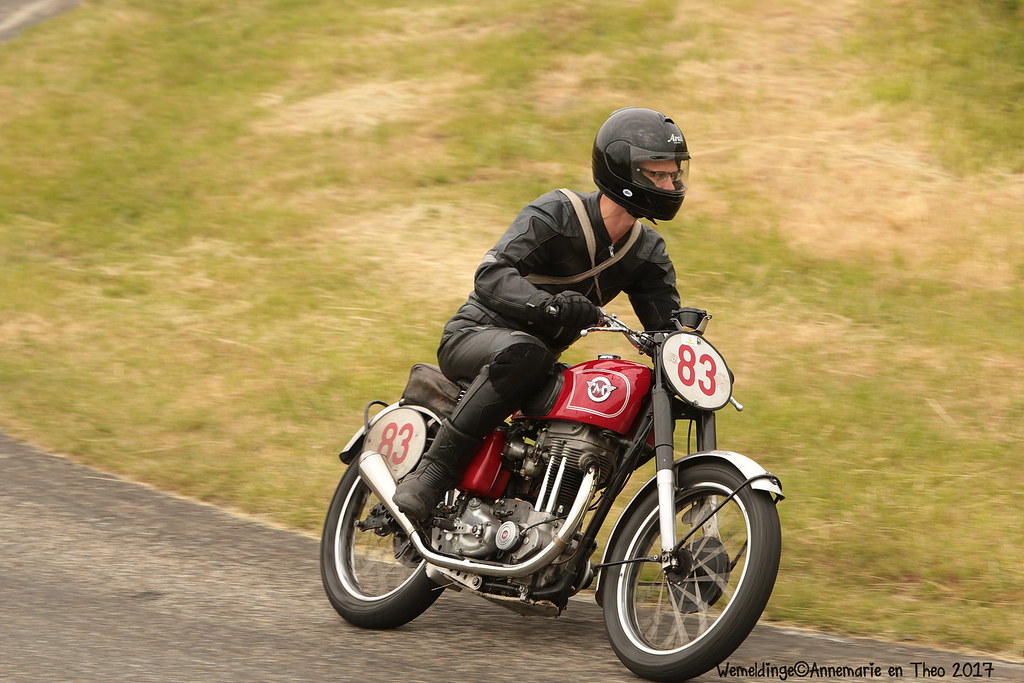The image captures an action-packed moment of a man riding a motorcycle, potentially in a race, characterized by the number 83 in red within a white circle prominently displayed on the motorcycle's front and rear. The rider, clad entirely in black with a leather jacket, pants, boots, and gloves, is also protected by a black helmet with a clear visor under which he wears glasses. Adding to his gear is a beige backpack with straps crossed at the chest. He expertly maneuvers the red motorcycle with black accents and chrome pieces, including the exhaust and wheel spokes, that show a blur due to the rapid motion. The scene unfolds on a paved, winding road surrounded by green grass, hinting at an oval circuit. A portion of the road reappears in the top left corner, reinforcing the racing theme, and the image is dated 2017 in the bottom right corner.